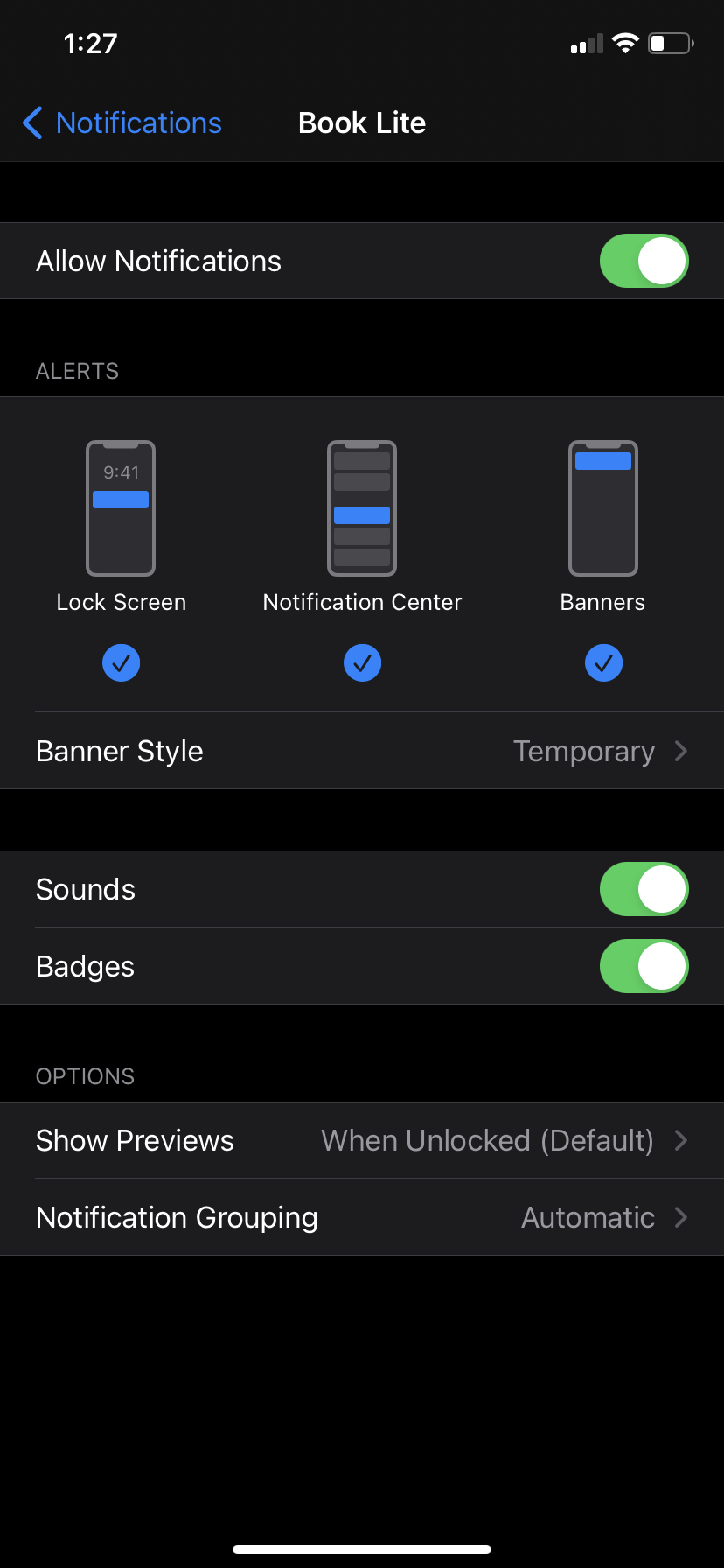The image showcases a screenshot from an iPhone displaying the notification settings page for an app called "Book Light." The user interface is consistent with the typical iOS design. At the top, there's an active toggle switch for "Allow Notifications," highlighted in green. Directly below, there are options for enabling alerts on the Lock Screen, Notification Center, and Banners. The banner style is set to "Temporary." The settings for "Sounds" and "Badges" are also active, indicated by their corresponding green toggles.

Toward the bottom, there are additional options listed under "Options." The first is "Show Previews," set to "When Unlocked (Default)." The second option, "Notification Grouping," is set to "Automatic." This settings page offers comprehensive control over the notification preferences for the Book Light app, which appears to be an e-book reader application.